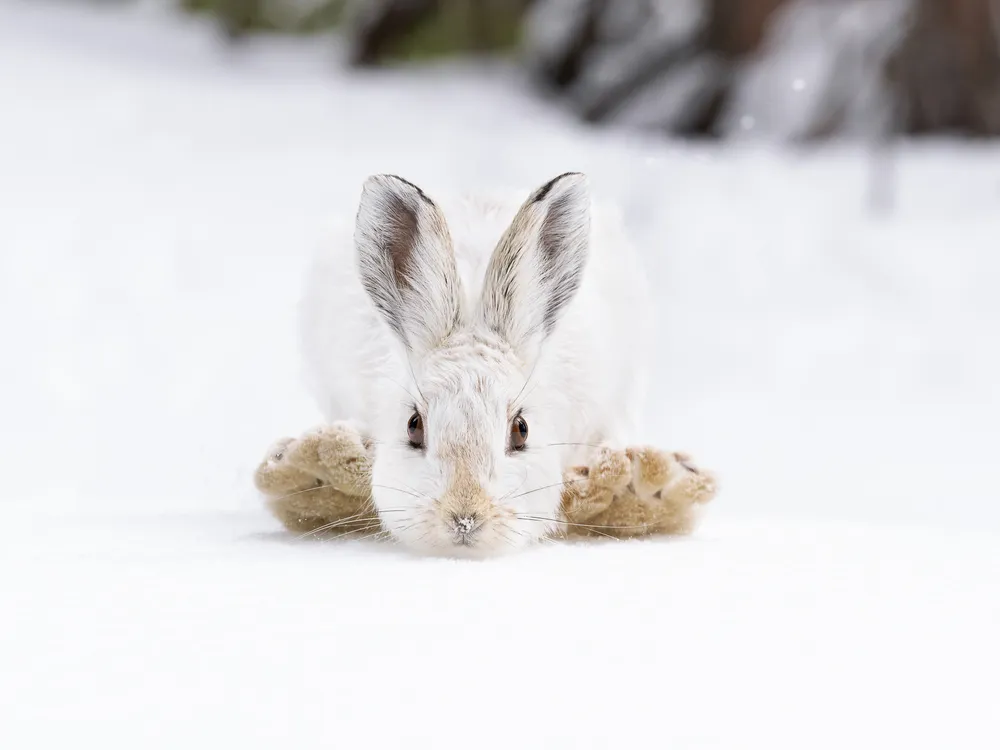In this image, a small white rabbit is nestled into a snowy landscape, its head resting on something brownish that resembles a sponge. The rabbit's big, dark eyes gaze toward the camera while its long, fluffy ears, tinged with darker shades, stand upright. The foreground showcases the intricate detail of the snow-covered ground where it lies. In the background, the whiteness of the snow gradually blurs into a scene where indistinct shapes suggest the presence of trees or rocks, adding an enigmatic charm to the overall wintery setting.